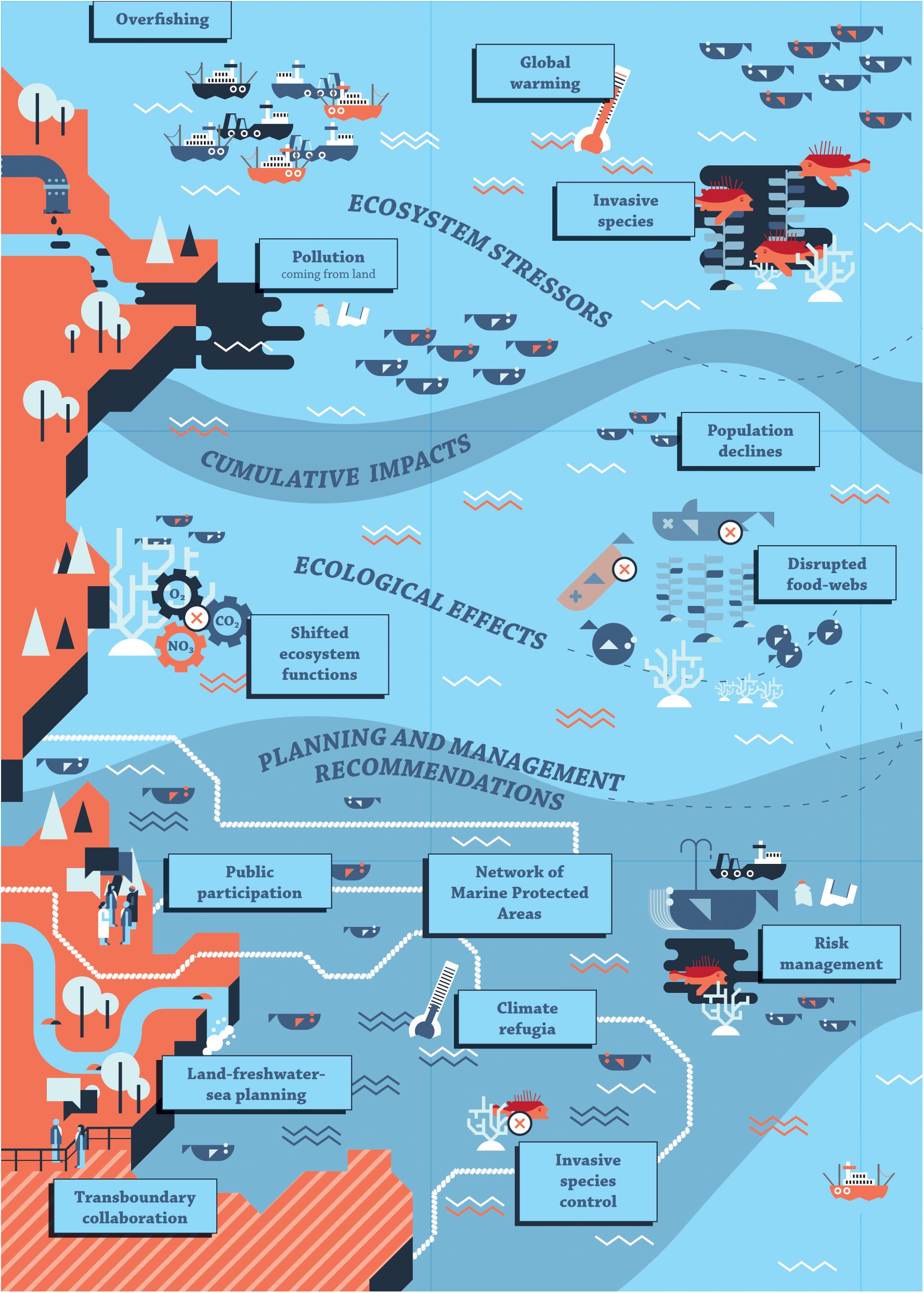The image is a detailed, cartoon-like infographic on a light blue background, illustrating the various stressors affecting ocean ecosystems, their ecological impacts, and potential solutions. On the left side of the poster, an orange rectangular area represents land, transitioning into a bluish area depicting the ocean. 

At the top left, there is a graphic of overfishing represented by small boats, alongside a text box labeled "Overfishing." Below this, an illustration indicates pollution emanating from land, marked by a black blob. Further to the right, red spiny fish signify invasive species, with a corresponding text box. At the very top, a thermometer icon highlights the issue of "Global Warming."

Central to the infographic is the overarching theme of "Ecosystem Stressors" with various text boxes elaborating on cumulative impacts. These stressors lead to significant ecological effects such as "Population Declines," "Disrupted Food Webs," and "Shifted Ecosystem Functions."

Toward the bottom, the infographic proposes planning and management solutions, each in blue rectangles with corresponding icons. The recommendations include "Public Participation," "Network of Marine Protected Areas," "Climate Refuge," "Risk Management," "Invasive Species Control," "Land, Freshwater, and Sea Planning," and "Transboundary Collaboration."

Overall, the infographic effectively conveys the complex issues facing ocean ecosystems due to stressors like overfishing, pollution, global warming, and invasive species, and suggests comprehensive strategies for addressing these challenges.